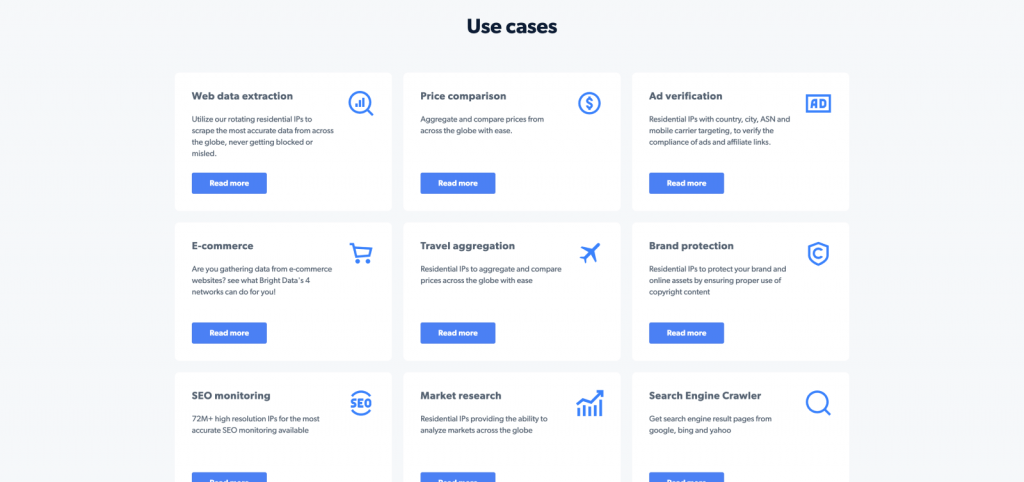The image depicts a website that outlines various use cases at the top. Underneath, it features nine different selections organized in a three-by-three grid layout. Each selection pertains to a specific service, and they include brief descriptions along with a "Read More" option for further details.

In the first row:

1. **Web Data Extraction**: Describes utilizing rotating residential IPs to extract the most accurate global data, ensuring the process is never blocked or misled.
2. **Price Comparison**: Highlights the ability to aggregate and compare prices from around the world with ease.
3. **Ad Verification**: Explains targeting residential IPs with country, city, ASN, and mobile carrier specifics to verify the compliance of ads and affiliate networks.

In the second row:

4. **eCommerce**: Mentions the utility of gathered data from eCommerce websites and discusses what the right data network can do for users.
5. **Travel Aggregation**: Focuses on using residential IPs to aggregate and compare travel prices globally, again emphasizing ease.
6. **Brand Protection**: Discusses using residential IPs to protect brand and online assets by ensuring the proper use of copyrighted content.

In the third row:

7. **SEO Monitoring**: With a database of over 82 million high-resolution IPs, provides the most accurate SEO monitoring available.
8. **Market Research**: Describes residential IPs capabilities in analyzing global markets and errors.
9. **Search Engine Crawler**: Details obtaining search engine result pages from major search engines like Google, Bing, and Yahoo.

Each service offers a "Read More" button to explore further details. The layout and concise, informative descriptions make it easy to understand the wide range of applications these services provide.